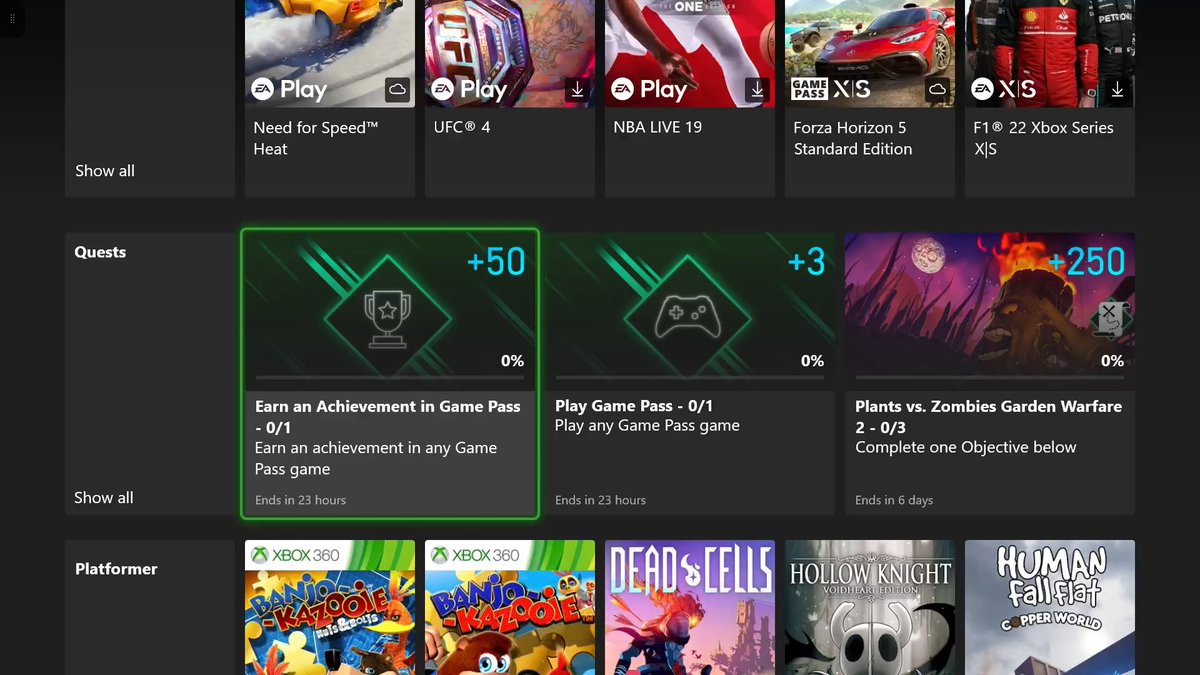The image showcases a digital gaming dashboard on an Xbox Series X|S console, highlighting various game titles and challenges. Featured prominently are games such as "Need for Speed: Heat," "UFC 4," "NBA Live 19," "Forza Horizon 5 (Standard Edition)," "F1 22," and "Plants vs. Zombies: Garden Warfare 2." The dashboard displays several active quests and achievements to be earned through the Xbox Game Pass service. One quest requires players to earn an achievement in any Game Pass game, with a progress indicator showing "0 to 1." Another objective challenges players to play any Game Pass game, with a timer indicating it ends in 23 hours. Additionally, there is a quest labeled "Show All," which likely refers to viewing all available quests, along with specific objectives such as completing one listed challenge within 6 days and other achievements offering in-game rewards like "plus 50," "plus 3," and "plus 2."